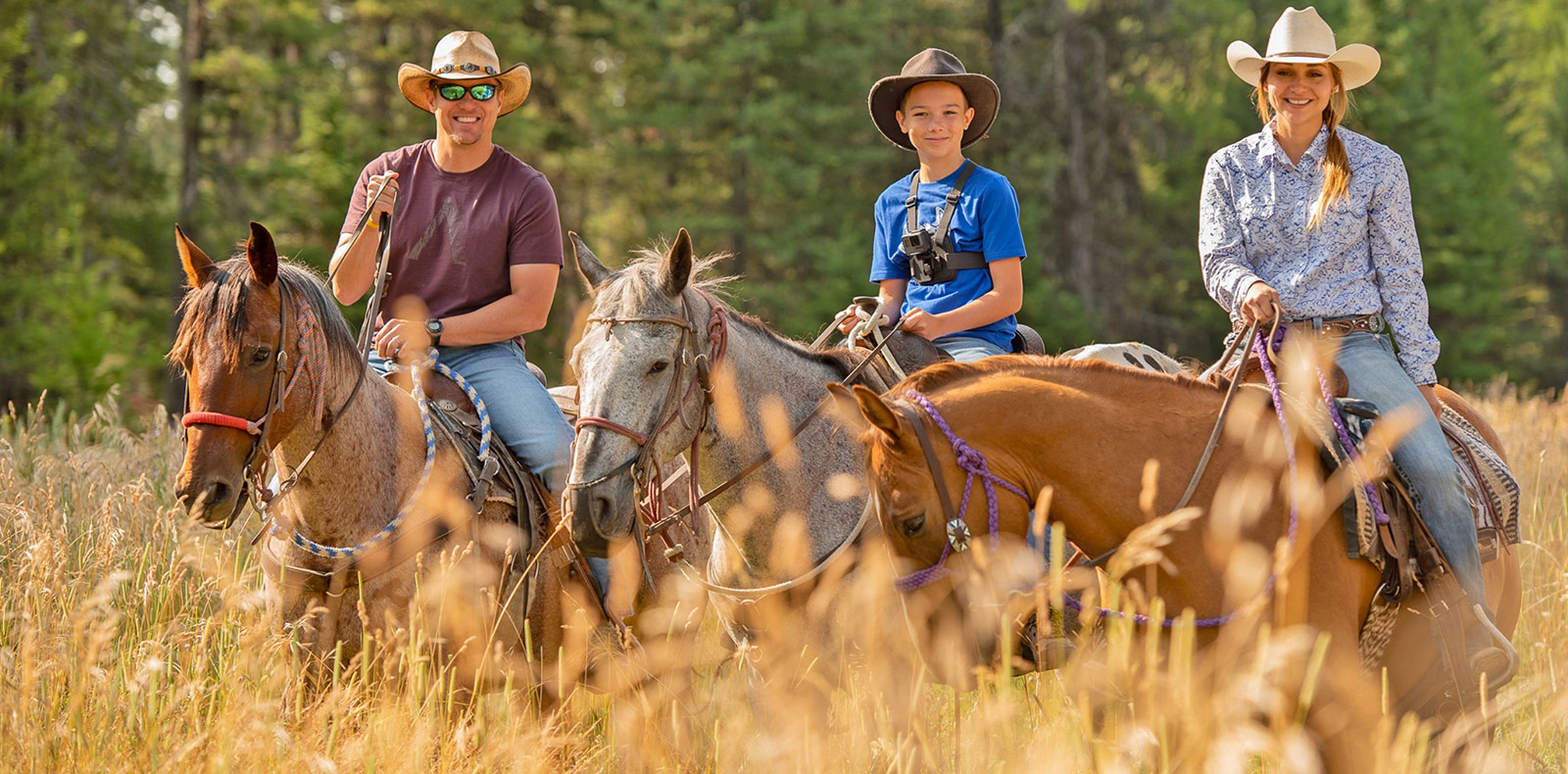In this charming outdoor family portrait, three family members are captured sitting atop three different horses, smiling warmly at the camera on a sunny day. They are positioned closely together in a field of tall, dried, wheat-like grass with a dense tree line of evergreen trees filling the background. 

To the left is the father, dressed in blue jeans, a mauve-purple crew neck t-shirt, a cowboy hat, and sunglasses. He sports a toothy smile and a wristwatch. His horse is a striking red roan with a grayish mane and tail. In the middle is the young son, likely around 12 years old, seated on a fleabane gray horse. He is wearing a blue t-shirt, blue jeans, and a gray felt hat, with a GoPro camera strapped to his chest, reflecting his adventurous spirit. 

On the right, the mother sits gracefully on a dun or sorrel horse. Her attire includes blue jeans, a brown belt, a long-sleeve blue and white floral shirt, and a tan cowboy hat, with her hair pulled back in a braid. This heartfelt image likely captures a family moment in a peaceful meadow, united by their shared passion for horseback riding.